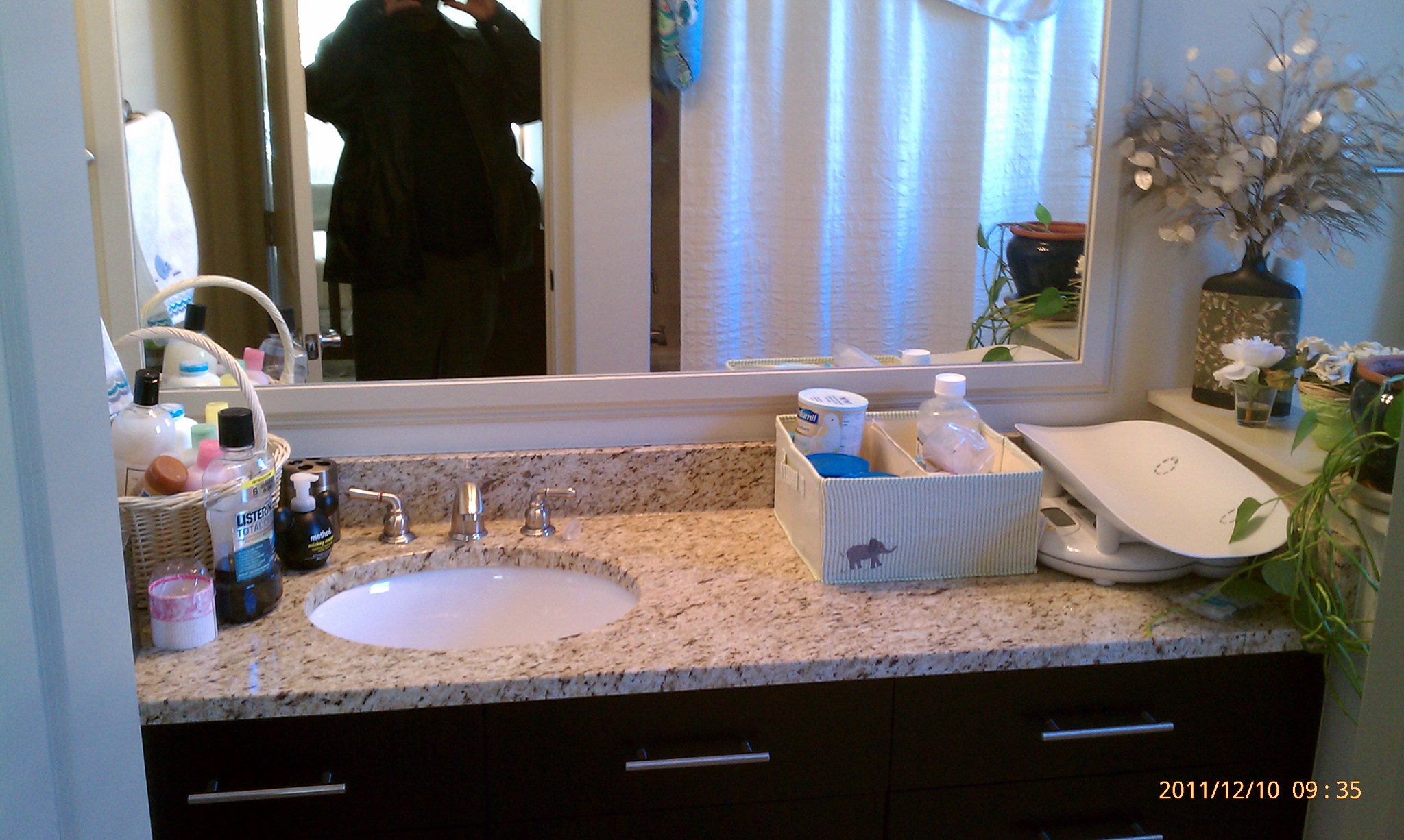This photograph captures the interior of a home bathroom, dated December 10th, 2011 at 9:35 AM. The bathroom features a granite countertop with a single sink, equipped with chrome faucets and handles. An off-white shower curtain conceals the shower area. A half-wall hosts a vase with dried dollar plants, a planter with a vibrant spider plant, and a glass containing a flower and possibly other faux flowers. 

The countertop is adorned with various items, including a fabric box containing infant supplies, a small white baby scale, a basket with lotions, a bottle of Listerine, and a pump bottle of hand soap. The vanity is constructed from brown wood. The mirror's reflection reveals a person dressed in a black top and pants, taking the photo.